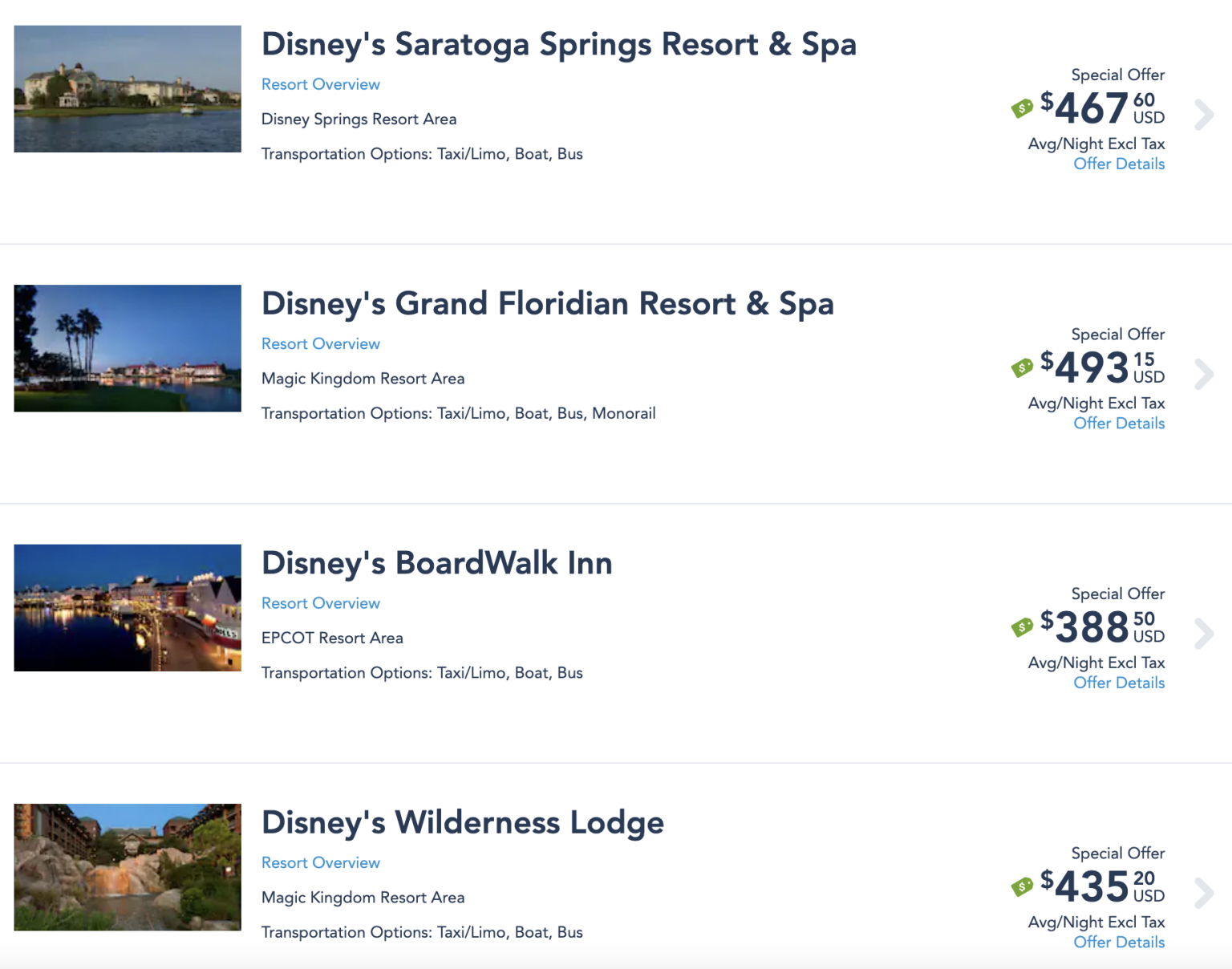This image showcases a screenshot of a search for Disney hotels, featuring four distinct options:

1. **Disney's Saratoga Springs Resort & Spa**:
   - **Visual Description**: A beige-colored, elongated hotel situated by a serene lake with a vehicle or watercraft visible on the lake’s surface. The backdrop features a clear blue sky.
   - **Text Details**: 
     - "Disney’s Saratoga Springs Resort & Spa"
     - "Resort Overview" (clickable, in blue)
     - "Disney Springs Resort Area"
     - "Transportation Options: Taxi/Limo, Boat, Bus"
     - "Special Offer" (highlighted with a green tag): "$467.60 USD average/night (excluding tax)"
     - "Offer Details" (clickable, with a right-pointing caret)

2. **Disney's Grand Floridian Resort & Spa**:
   - **Visual Description**: A picturesque hotel adjacent to a lake, complemented by palm trees and expansive green areas.
   - **Text Details**:
     - "Disney’s Grand Floridian Resort & Spa"
     - "Resort Overview" (clickable, in blue)
     - "Magic Kingdom Resort Area"
     - "Transportation Options: Taxi/Limo, Boat, Bus, Monorail"
     - "Special Offer" (highlighted with a green tag): "$493.15 USD average/night (excluding tax)"
     - "Offer Details" (clickable, with a right-pointing caret)

3. **Disney's Boardwalk Inn**:
   - **Visual Description**: Various hotels are situated along a large river or body of water next to a boardwalk.
   - **Text Details**:
     - "Disney’s Boardwalk Inn"
     - "Resort Overview" (clickable, in blue)
     - "Epcot Resort Area"
     - "Transportation Options: Taxi/Limo, Boat, Bus"
     - "Special Offer" (highlighted with a green tag): "$388.50 USD average/night (excluding tax)"
     - "Offer Details" (clickable, with a right-pointing caret)

4. **Disney's Wilderness Lodge**:
   - **Visual Description**: The image highlights a rustic-looking hotel designed to resemble a cabin, surrounded by large boulders and greenery with a water feature and rocky terrain in the background.
   - **Text Details**:
     - "Disney’s Wilderness Lodge"
     - "Resort Overview" (clickable, in blue)
     - "Magic Kingdom Resort Area"
     - "Transportation Options: Taxi/Limo, Boat, Bus"
     - "Special Offer" (highlighted with a green tag): "$435.20 USD average/night (excluding tax)"
     - "Offer Details" (clickable, with a right-pointing caret)

The screenshot neatly presents the essential information for each hotel, including visual appeal, various amenities, and special offers.